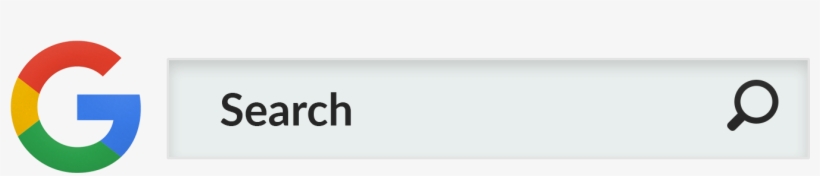This image features the iconic multi-colored Google logo prominently displayed in the center. The "G" of the logo starts at the top with red, transitions into a small segment of yellow, followed by a longer green section, and finally culminates in a blue corner that forms the angular end of the "G." Below the logo is a search bar, which contains the word "Search" in gray text. To the right of the text, there is a magnifying glass icon, symbolizing the search function. The rest of the page is blank, accentuating the simplicity and focus of the design. The image was likely captured in Bluetooth mode.